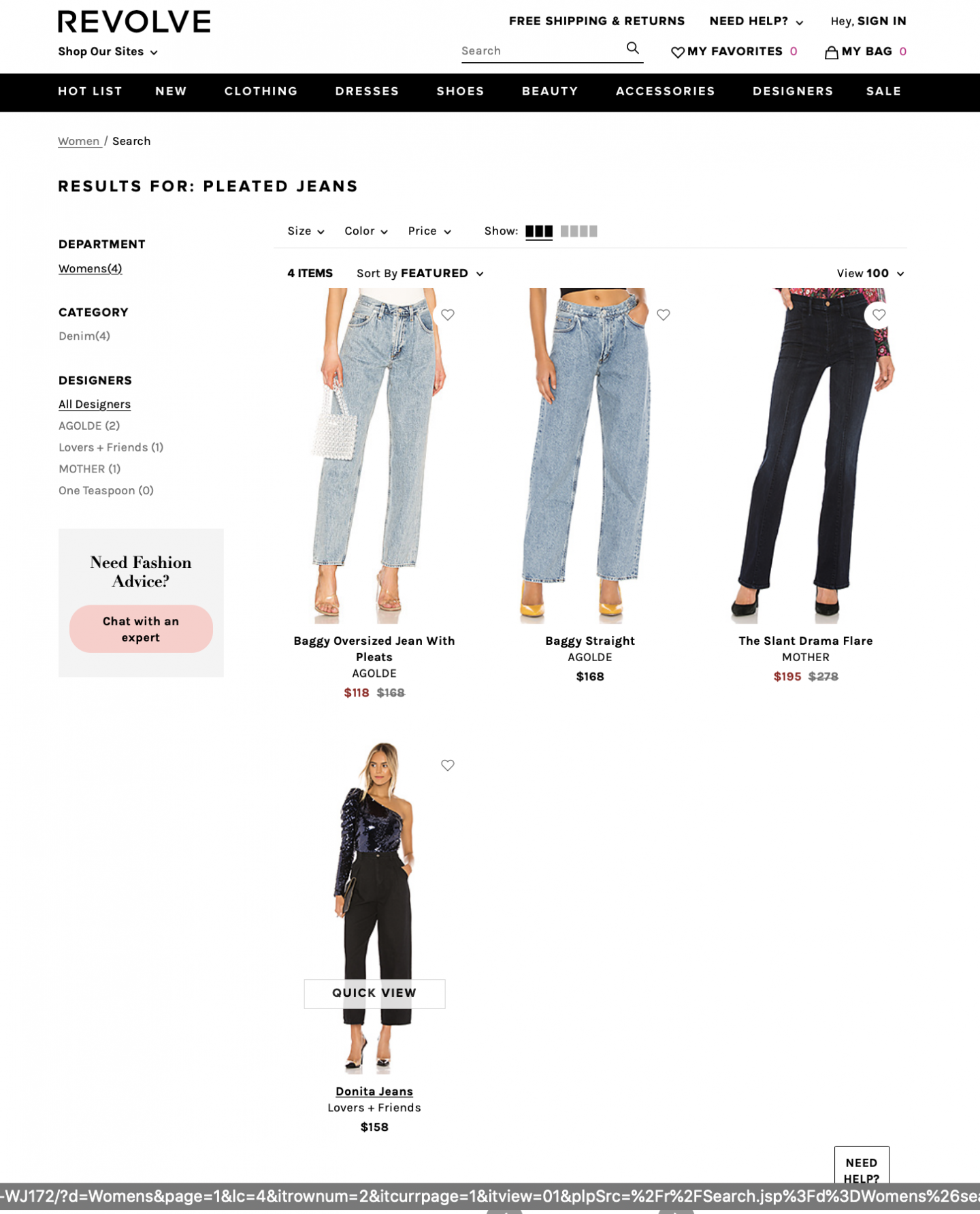We are currently browsing the Revolve shopping website, which offers a range of women's jeans. Featured prominently are four pairs of pleated jeans, each with a cropped length that reveals the ankle. The selection includes two black and two blue jeans, priced between $118 and $195. This price range is considered moderate in today's market, though it doesn't necessarily guarantee high quality.